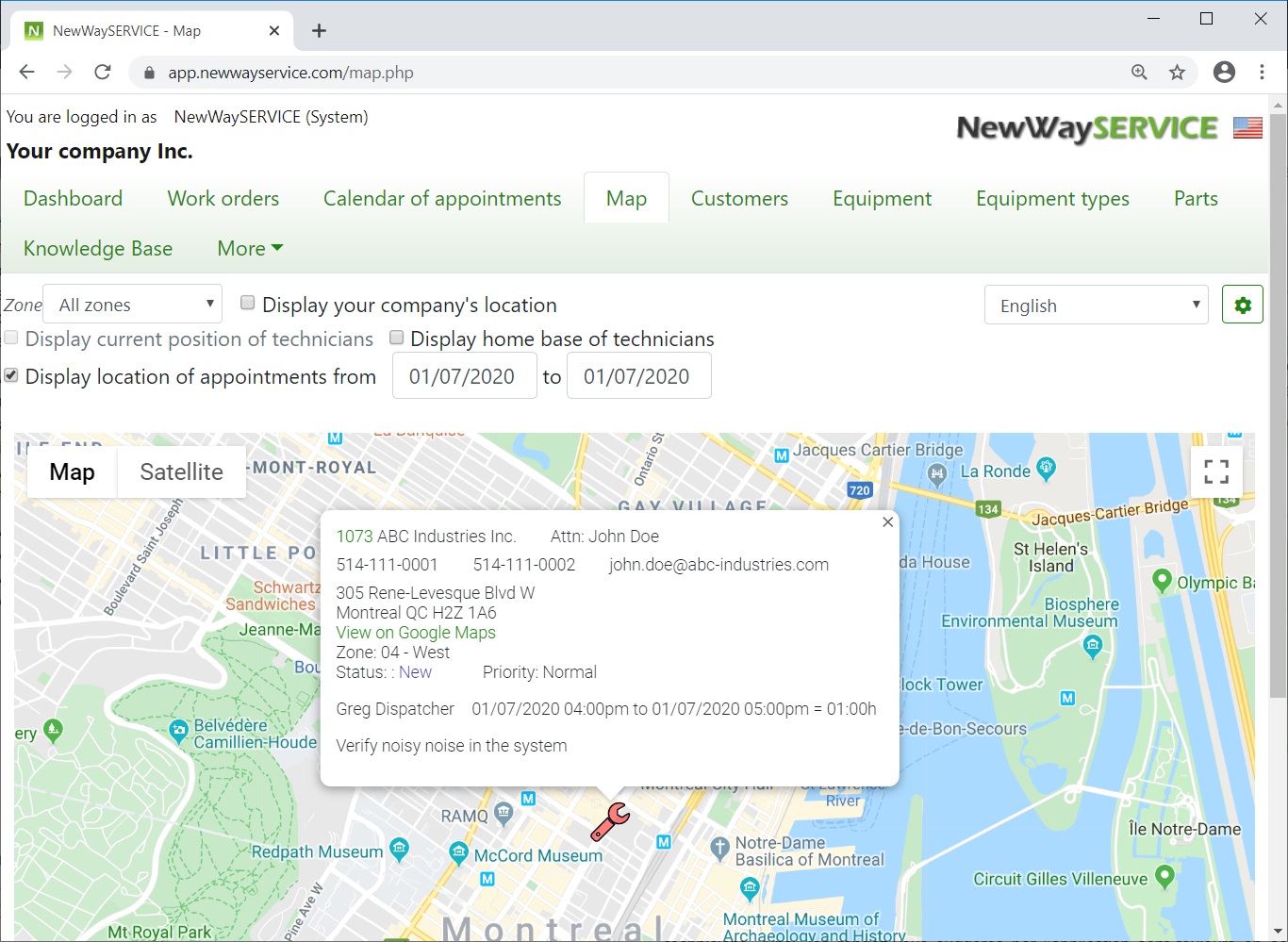Here is a detailed and cleaned-up version of the caption:

---

The image showcases a webpage from New Way Service, an application accessible via the URL app.newwayservice.com/map.php. At the top of the interface, it prominently displays "New Way Service - Map." The user is logged in under the name "New Way Service" with the indicator "system." The sidebar menu, color-coded in a faint green, lists several navigation options in green print: Dashboard, Work Orders, Calendar of Appointments, Map, Customers, Equipment, Equipment Types, Parts, Knowledge Base, and more.

At the top of the sidebar, the application logo reads "NewWay" (all in black letters) followed by "SERVICE" (all in uppercase green letters). Further down, the user can select "Zones" with the current selection set to "All Zones for display." 

The main section of the page features a map displaying the company's location, with various markers. One notable marker, shaped like a wrench, is associated with the task "Verify noisy noise in the system," specifically addressed to "Attention John Doe," prominently displayed on the lower part of the map.